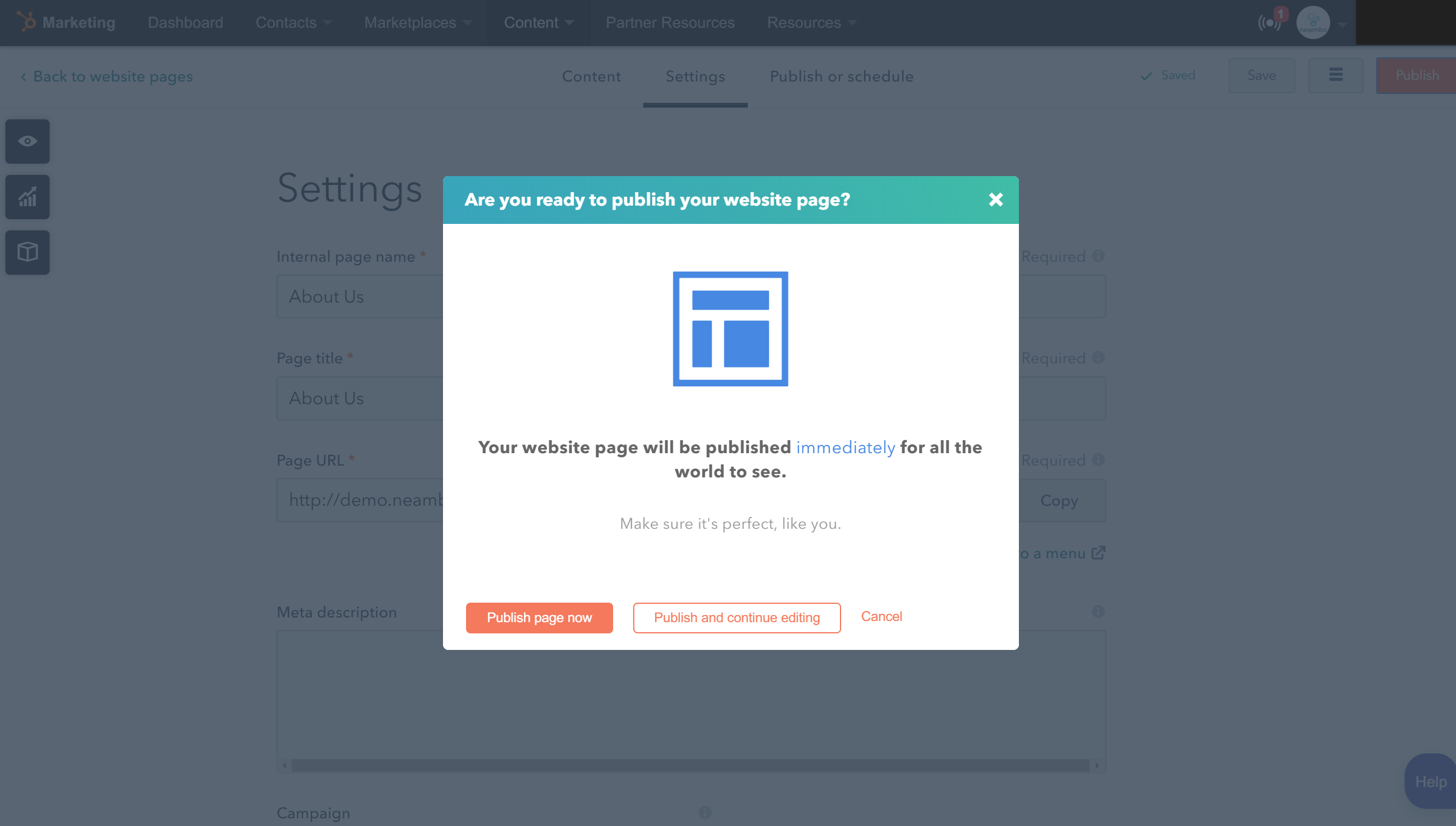The image displays a grey-themed user interface featuring numerous sections and action items. 

At the top, there's a header with tabs labeled "Marketing," "Dashboard," "Contacts," "Marketplaces," "Content," and "Partner Resources." On the left side of the screen, a sidebar presents a navigation menu with options such as "Back to WhatsApp Pages," an icon labeled "Hot," "Grab," "Queue," "Content," "Settings," "Publisher Schedule," "Internal Page," "Name," "Star," "About Us Page Title," "About Us Page URL," and "Description."

The main window prominently displays a message, "Are you ready to publish your WhatsApp page?" just beneath the top part of the screen. Below this message, a blue bar contains grey-colored text stating, "Your WhatsApp page will be published immediately for all the world to see. Make sure it’s perfect like you." Adjacent to this, there are three action buttons: "Publish Page Now" and "Publish and Continue Editing" are centrally located, while the "Cancel" button is towards the right.

In the upper-right corner, the screen maintains the grey color scheme, while a noticeable red square button with blue edges is labeled "Publish." Additionally, there's a section denoted as "Help" for user assistance.